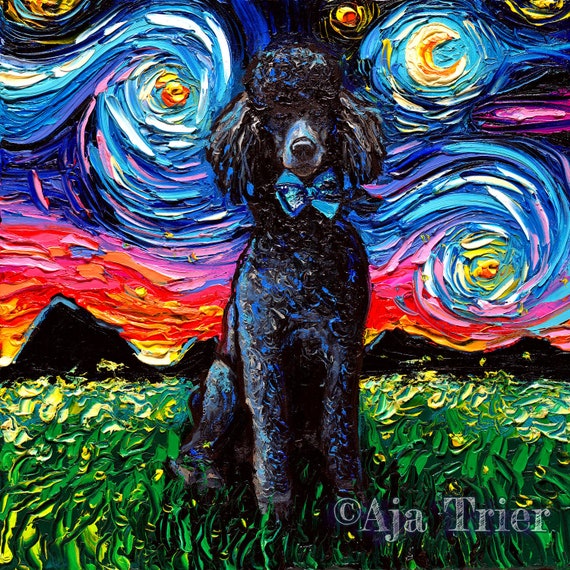This vibrant oil painting captures a black poodle, reminiscent of Vincent van Gogh's Starry Night in style. The poodle, distinguished by its curly hair and adorned with a blue bow tie, sits attentively in a field of green grass, gazing directly at the viewer. The background showcases a whimsical sky filled with blue and yellow swirling patterns, echoing van Gogh’s iconic aesthetics. Above the dark, undulating mountains, the sky transitions from evening hues of orange and yellow near the horizon to deeper blue and purple tones dotted with swirling clouds. Notably, a crescent moon is integrated into the swirling sky, adding a touch of ethereal beauty to the scene. The bottom right corner of the painting features a watermark indicating © Aja Trier, the artist.